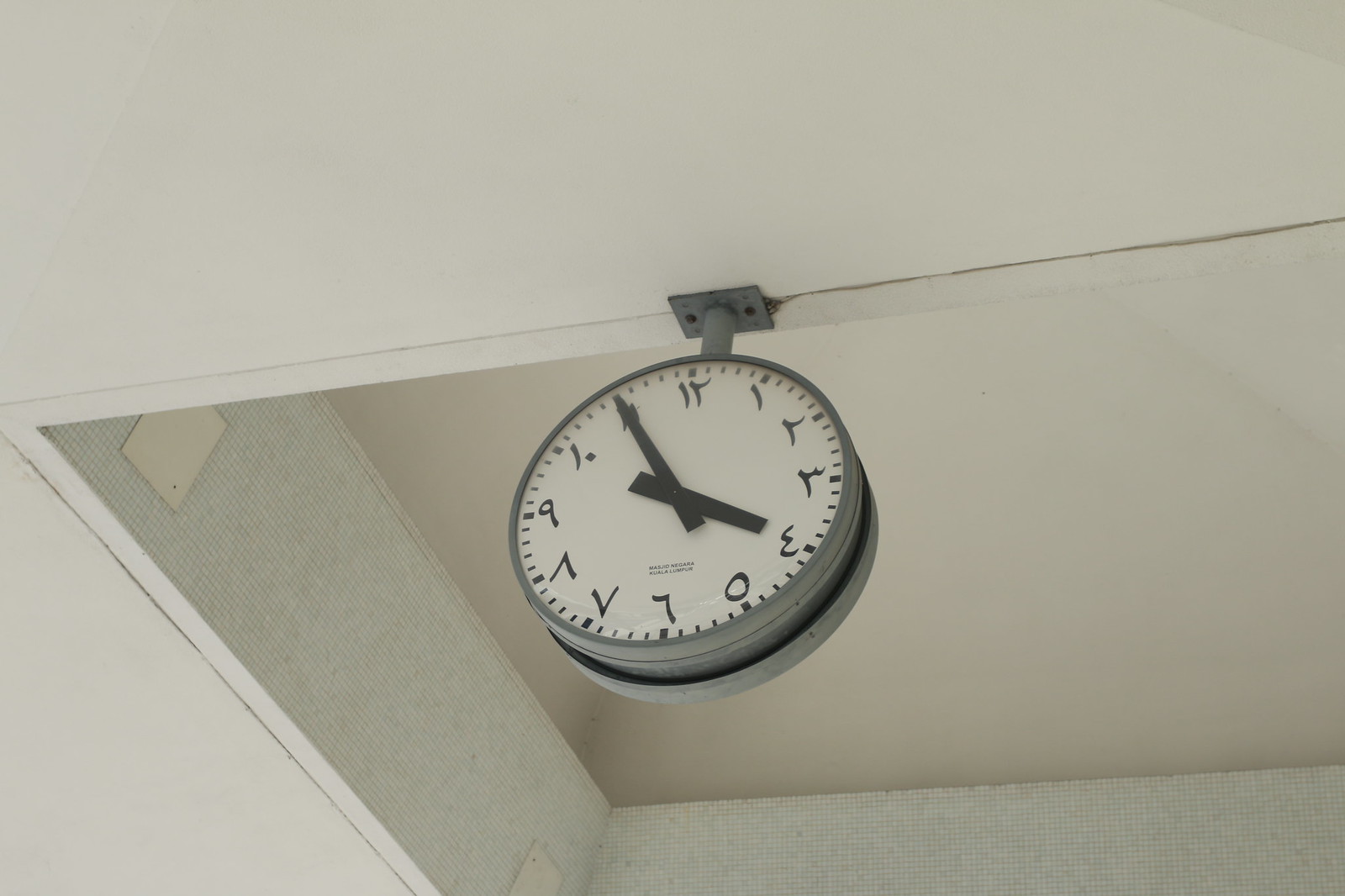This image captures a centrally-placed wall clock hanging from a ceiling bracket in a white-ceilinged room. The clock, framed by a gray outer circle and featuring a white inner circle, displays an unusual numeral system that differs from traditional English or Roman numbers. Its minute and hour hands are black. Above the clock, the white ceiling has a cutout, possibly resembling a skylight, that is off-centered and extends from the lower edge to the upper portion of the ceiling. Additionally, there are two square white markers on the ceiling near the clock, adding to the architectural detail of the room.